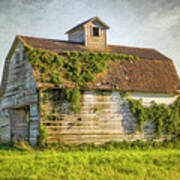This photograph, taken outdoors on a cloudy, possibly rainy day, showcases a large, dilapidated wooden barn covered in vibrant green moss and ivy. The aged structure features planks that are peeling away with visible holes, giving it a very rustic and weathered appearance. The barn has a brown to red-colored roof, also showing signs of aging, with plants growing all over it. An open loft window is situated towards the top of the barn, which adds to its rustic charm. Thick, vibrant green grass grows in the foreground, contrasting with the muted tones of the barn’s weather-beaten facade. The sky above is a dark, muted gray, enhancing the somber, abandoned feeling of the scene.